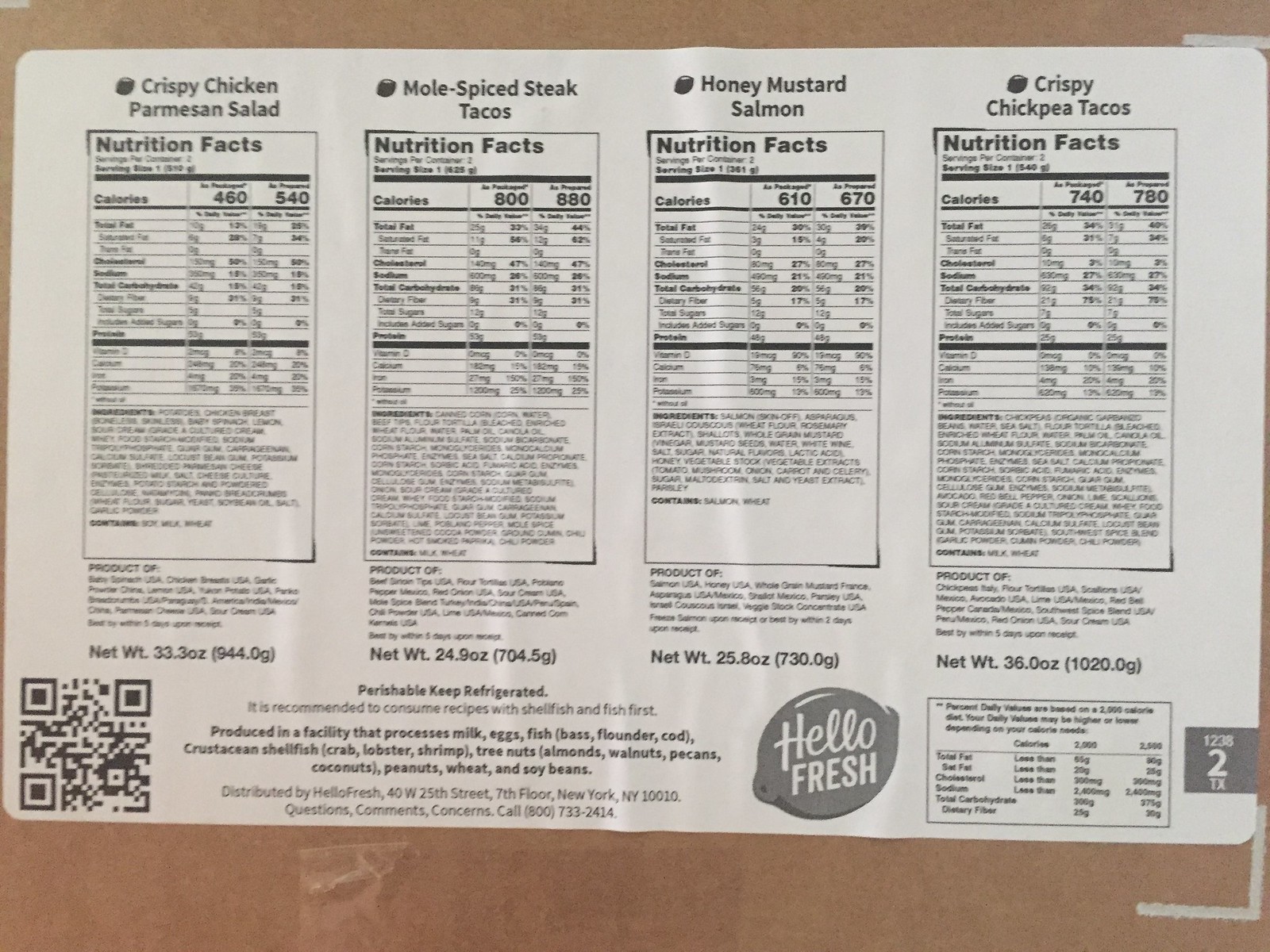The image captures a cardboard box with a large white label prominently displayed on its side, adorned with the HelloFresh logo and a lemon emblem in a gray oval toward the bottom center-right. The label includes four panels detailing the nutritional information for different meal kits: Crispy Chicken Parmesan Salad, Mole Spiced Steak Tacos, Honey Mustard Salmon, and Crispy Chickpea Tacos. Each panel lists the respective calories for the packaged and prepared meals: 460 and 740 for the Crispy Chicken Parmesan Salad, 800 and 880 for the Mole Spiced Steak Tacos, 610 and 670 for the Honey Mustard Salmon, and 740 and 780 for the Crispy Chickpea Tacos. Each meal kit provides two servings per container. A note at the bottom advises keeping the contents refrigerated due to perishability and recommends consuming recipes containing shellfish and fish first. Additionally, there is a QR code in the bottom left corner and an address indicating the shipment originates from New York, New York. Reflective tape and subtle white lines are also visible on the cardboard box exterior.